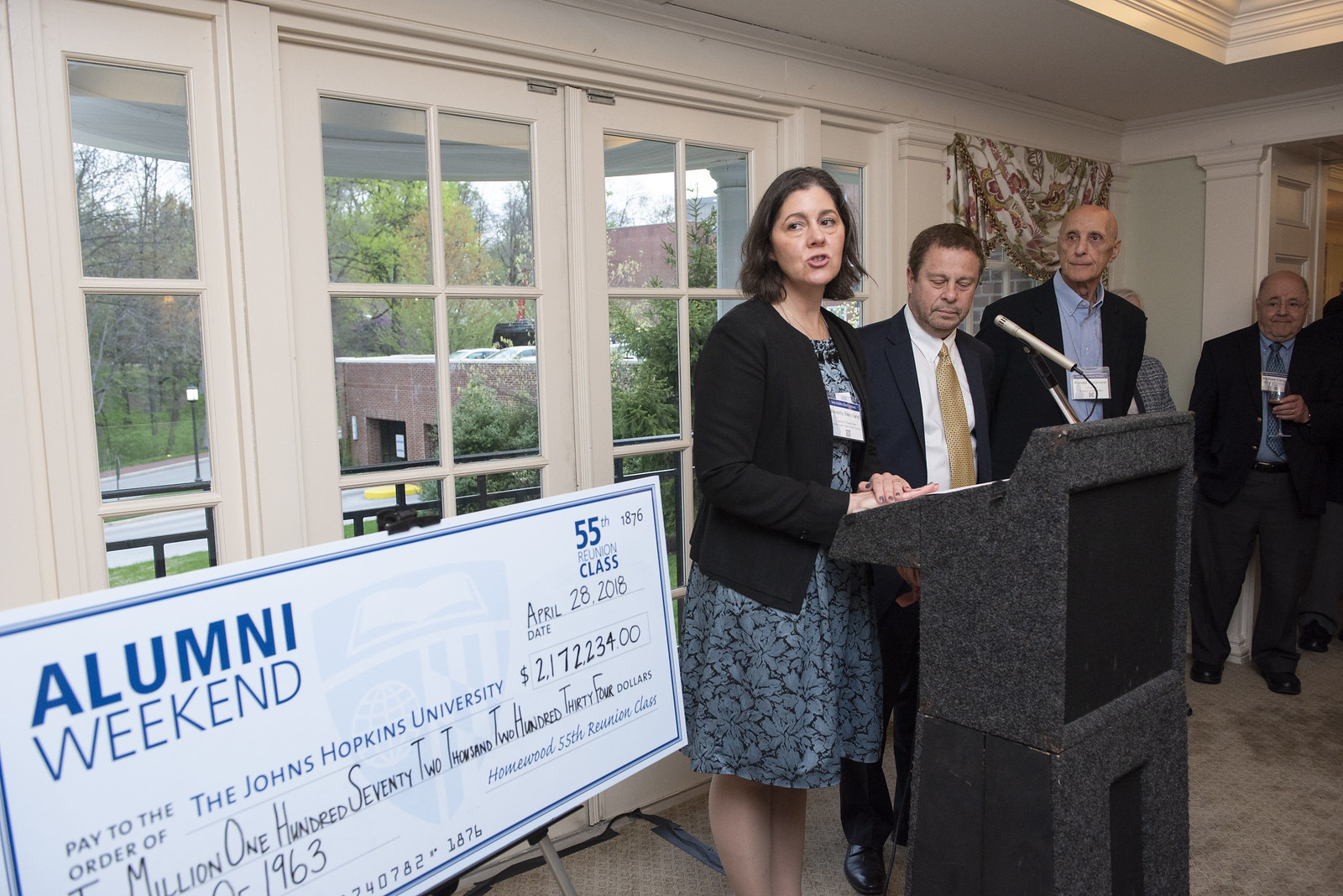A woman with shoulder-length black hair stands at a gray, square podium with a black square on its front, speaking into a silver microphone. She wears a blue dress with a long-sleeve black sweater over it and a lanyard with a name tag hanging in front of her. The event appears to be part of an Alumni Weekend celebration. Behind her is an enormous light blue check made out to Johns Hopkins University for $2,172,234, dated April 28, 2018. The check is marked from the 55th Reunion Class of 1963, with "Homewood" imprinted on the right-hand side. To her right stand three men in dark suits: the nearest man sports a gold tie, the next is a taller bald man wearing a light blue shirt without a tie, and the third is a shorter, older bald man in a dark suit with a blue shirt and tie, holding a wine glass. The background features French doors with glass panes, likely opening to a view of a college campus.